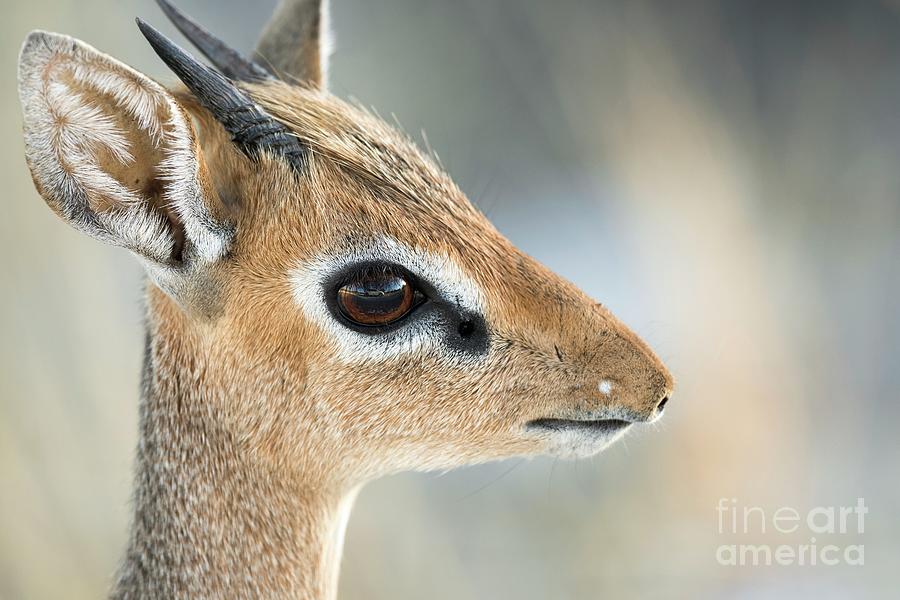This image is a close-up, side view of a Kirk's Dik-Dik, a small antelope native to Eastern Africa. It captures the animal in profile, facing the right, with a detailed focus on its head. The Dik-Dik has a distinct brownish-tan fur, similar to that of a white-tailed deer, but what sets it apart are its unique facial features. It has a thin neck and large, expressive brown eyes with a prominent white line around each. Notably, it has a narrow, almost mouse-like nose, different from the typical deer’s nose, giving it an unusual appearance.

The creature sports two small, straight, black horns positioned between its ears, which are also small and covered in white hair. The fur on its head transitions to a slightly darker tone towards the back of its neck. The background contrasts with the detailed subject, blending between dark and bright areas that are blurred, creating a focus on the animal itself. The image has a professional touch, indicated by the "Fine Art America" watermark in the lower right corner.